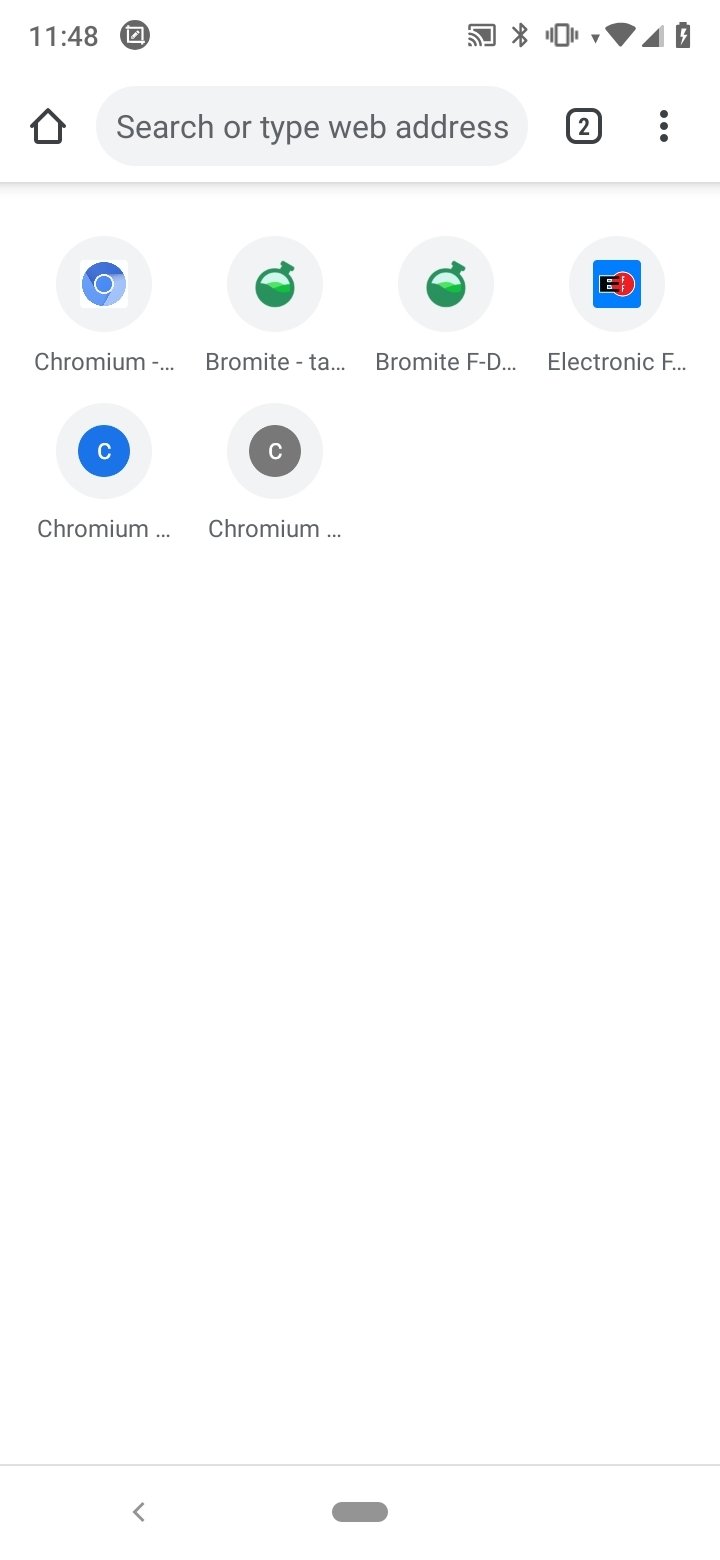A screenshot of a cell phone screen displaying a variety of UI elements and icons. The time reads 11:48 in the upper left corner. The right side of the status bar shows icons for Bluetooth, vibration, Wi-Fi, cellular signal strength, and a charging battery indicator below them. On the left side of the screen, there's a home icon followed by a search bar with the placeholder text "Search or type web address." Next to the search bar is a small box with the number "2" and a vertical ellipsis (three dots stacked vertically).

Below the search bar, there are two rows of app icons. The first row contains four icons labeled "Chromium," "Bromite," "Bromite-TA..." and "Bromite-FD..." The second row contains two icons, both labeled "Chromium..." The rest of the screen is blank, showcasing a minimalistic white background. 

At the bottom of the screen, there is a line, and below that, navigation elements: a left arrow, a thick bar in the middle, and some more colored indicators. The colors present in the interface include white, gray, blue, green, red, and black, on a predominantly white background.